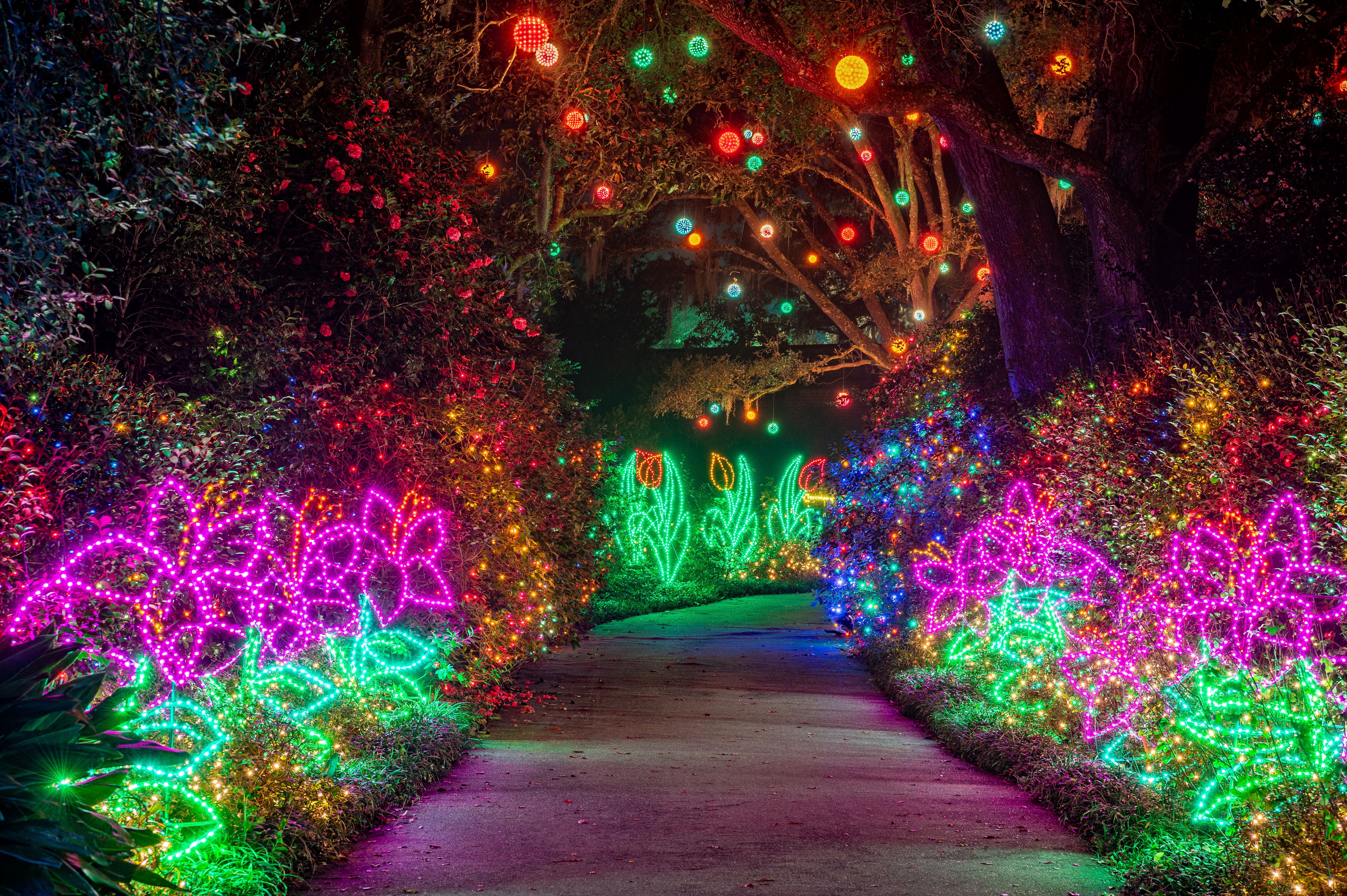This enchanted outdoor scene features a winding park walkway illuminated by an elaborate display of holiday lights, creating a mesmerizing, almost surreal atmosphere. The path, flanked by intricate light designs, is adorned with flowers crafted from lights, boasting pink petals and green leaves, reminiscent of daisies and tulips in red and orange hues. Larger green light shapes evoke the appearance of leafy foliage, interspersed with blue lights suggesting berries. The sidewalk reflects the vibrant pinks and greens of the lights, enhancing the ethereal glow. Above, large, round lights dangle from the branches, casting a magical canopy of light over the scene. Strings of multicolor lights meander through trees and bushes, some forming blossoms and designs, while others accentuate the natural contours of tall, cactus-like plants and small trees on either side of the path.